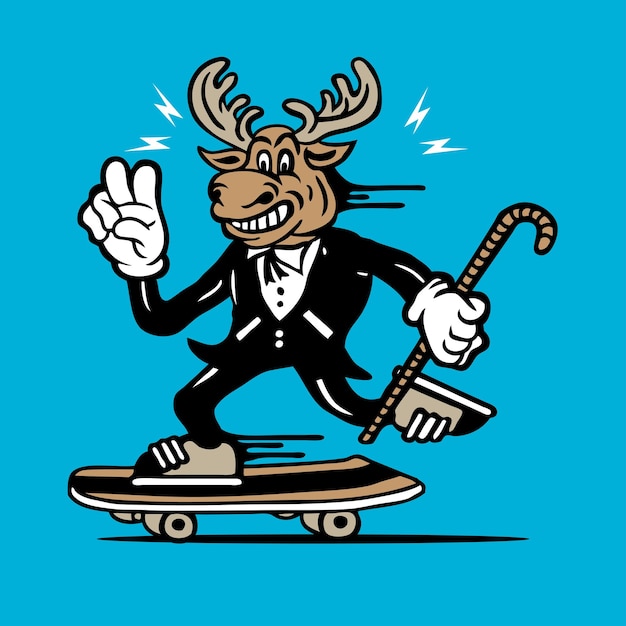The image depicts a highly stylized, computer-generated caricature of a moose character, likely based on Bow Winkle. The moose's head is a light brown color with tan antlers. It has a broad, cartoonish smile displaying numerous teeth and flared nostrils. Electrical bolts are seen around his antlers, enhancing his animated expression. The moose is adorned in a black tuxedo suit with a white button-up shirt and a bolo tie. He is wearing white gloves, with his right hand flashing a peace sign and his left hand holding a striped, light brown cane. The moose is balanced on a skateboard, featuring a light brown deck with a black stripe down the center and tan wheels. Additionally, he is wearing tan and black sneakers with white laces. The entire scene is set against a light blue or turquoise background, with motion lines indicating movement, giving a dynamic element to the modern, emoji-like illustration.